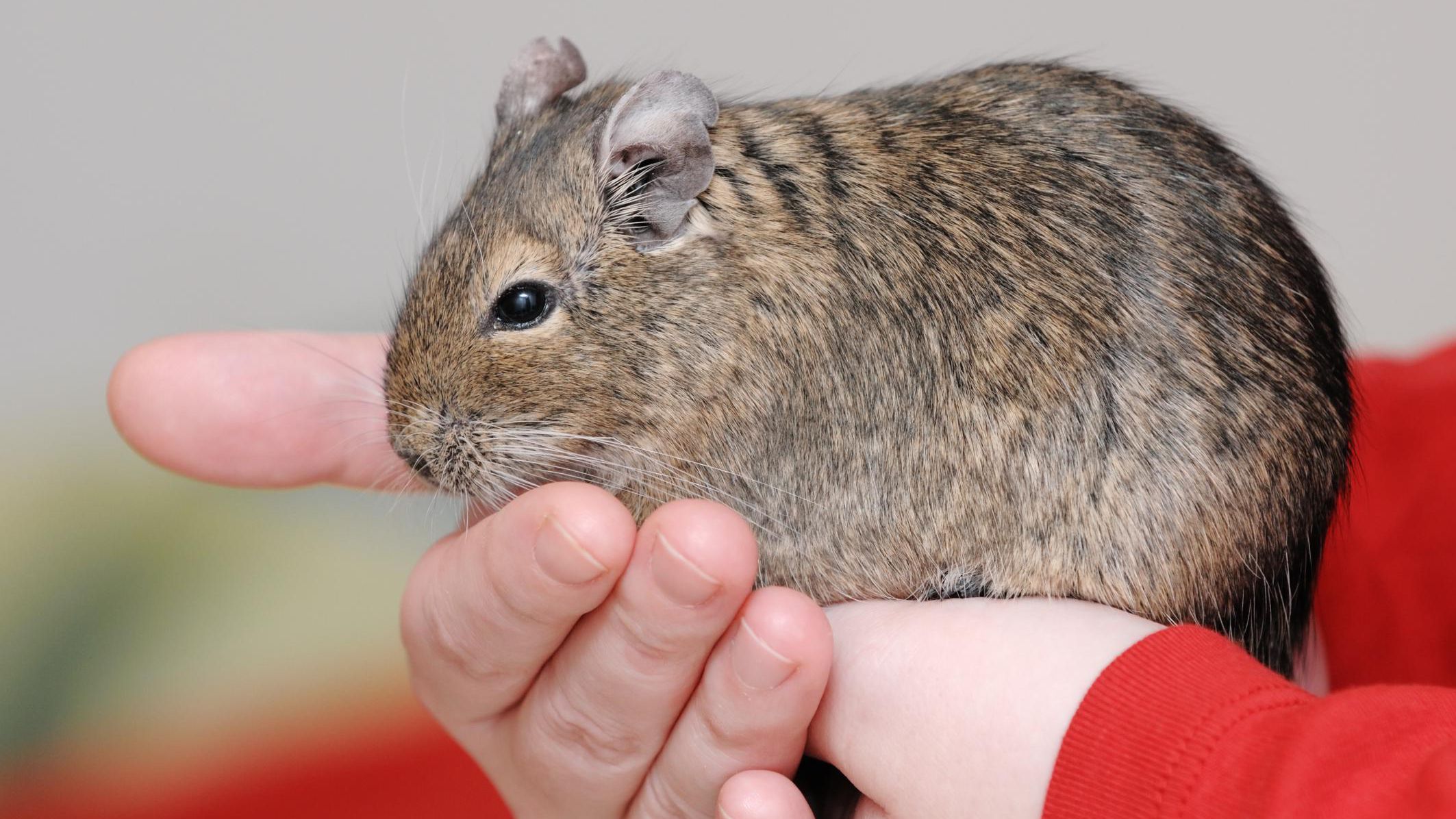This image captures an up-close view of a small rodent being gently held in a child's hands. The child's arms, clad in a long-sleeved red shirt, extend into the frame, their pale hands cupping the bottom and underside of the animal. The background is a softly blurred gray, which directs full attention to the rodent and the child’s hands.

The rodent, which appears to be a well-fed hamster, displays a mix of brown, black, tan, and gray colors throughout its body. Its coat is primarily brown and tan, with black and gray mingling, especially toward the back. It has small, rounded ears and a black nose with white whiskers protruding to each side. The animal's beady, black eyes reflect a sense of calm as it faces left, comfortably nestled in the child's gentle grip. The hamster's face is endearingly small, with nearly no visible neck, adding to its chubby, content appearance. This close-up highlights not only the adorable features of the hamster but also suggests the joy and safety a child might experience in holding such a pet.